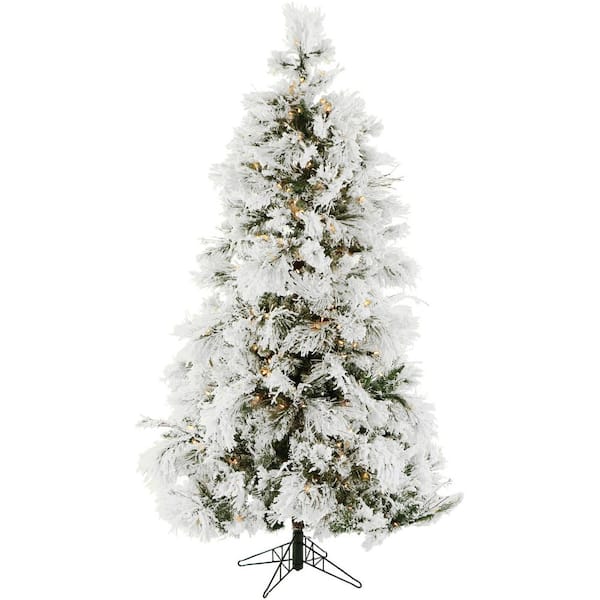This is a photograph of a medium-sized, artificial Christmas tree standing against a pure white background. The tree is supported by a black stand with four long, triangular prongs extending outwards in an X shape from the base. A black rod rises from the center to support the bulk of the tree. The tree itself is a typical evergreen, forming a perfect triangle with thick, dark green fronds that taper from a broad base to a narrow tip. The branches are densely coated in a white, powdery substance that mimics snow, clumping heavily along the edges of the tree and almost obscuring the underlying green. Dotting the tree are golden ornaments that peek through the thick layer of faux snow, although they are barely visible from certain angles. The tree is adorned with yellow lights placed at regular intervals, more noticeable where the green needles are exposed, adding a warm glow to its wintry appearance. Overall, the tree is pre-assembled and ready for display, capturing the essence of a snow-covered Christmas scene.